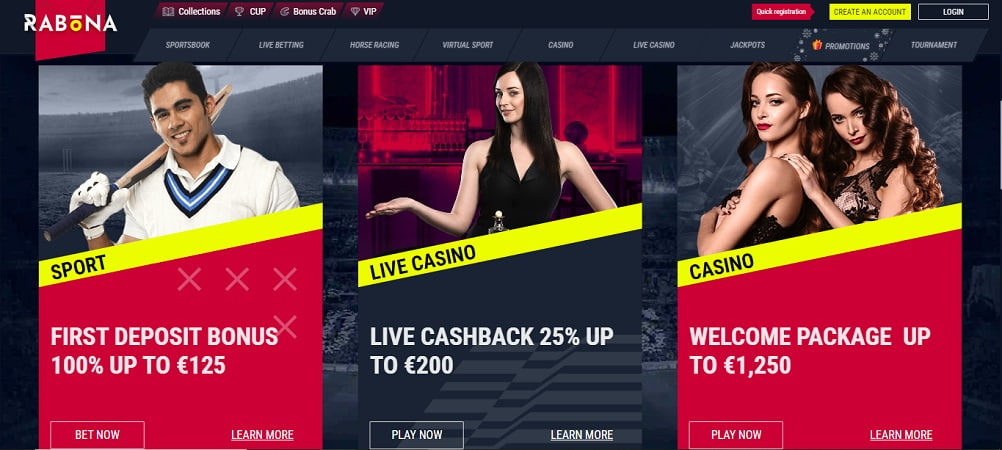This image is a screenshot of the homepage of the website Rabona. The website name "Rabona" is displayed prominently at the top, with the letters "R," "A," "B," "N," and "A" capitalized in white, while the "o" is in lowercase and colored yellow with a macron (a long line) above it, indicating its pronunciation. The navigation bar features sections for Collections, Cup, Bonus Crab, and VIP, as well as links to various gambling and gaming options including Sports Book, Live Betting, Horse Racing, Virtual Sport, Casino, Live Casino, Jackpots, and Promotions. In the upper right-hand corner, there is a yellow button labeled "Create an Account" and a red button for "Quick Registration." The main body of the page includes three distinct images: one of a man standing with a bat over his shoulder, another showcasing a live casino with a woman in a cocktail dress, and a third labeled "Casino" featuring two elegantly dressed women.